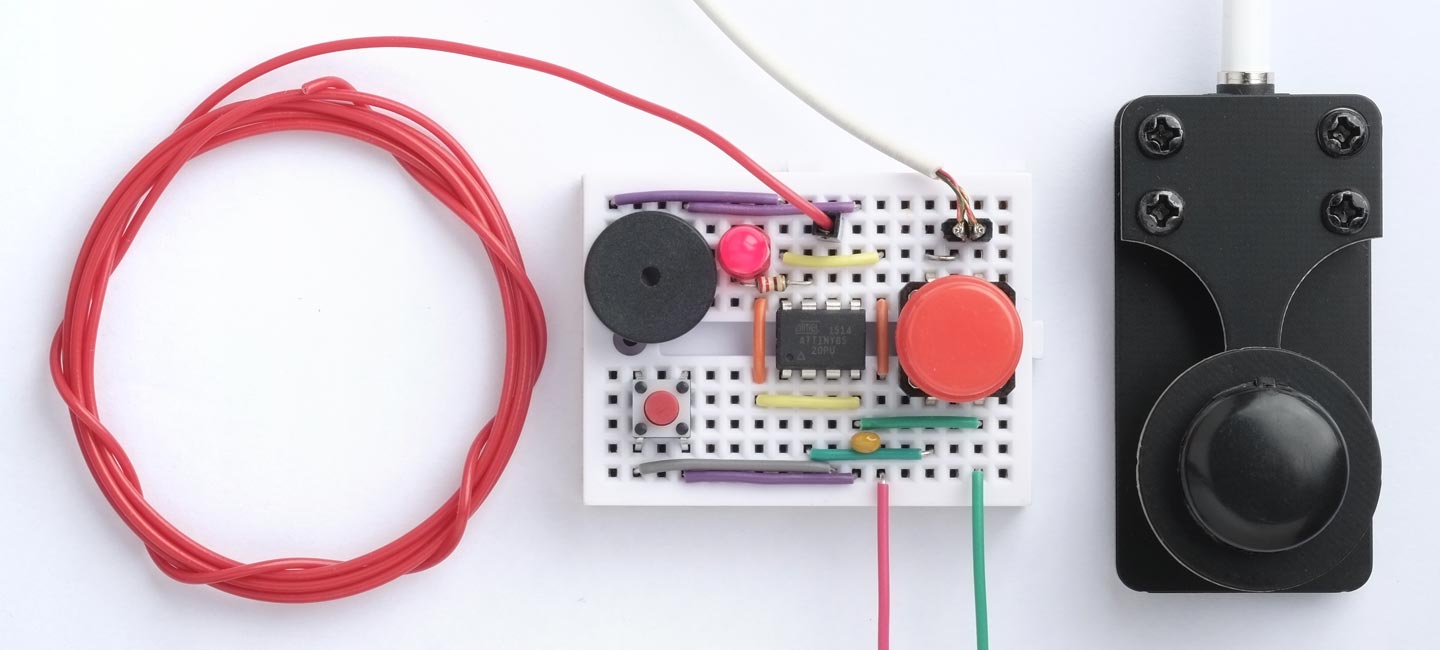The image showcases a detailed view of intricate electrical equipment that appears to be a homemade science project. The focal point is a circular arrangement of red electrical cords connected to a plate, from which several wires emanate. This plate features both a red cap and a black cap on opposite sides. It is intertwined with a green wire and a pink wire, as well as a white cord connected to an outlet at the top. Adjacent to this setup, a black rectangular electric component with rounded corners is visible, secured by four screws at its top corners and featuring a large round knob at the bottom. This component resembles an electric box. On the left, the image also contains a white plastic grid interwoven with purple and green wires, with various buttons and connectors—detail includes a red button and a black button, along with another small red button affixed with black elements, akin to small Lego pieces. This elaborate assembly of plastic and metal elements collectively appears to suggest some form of electrical process, possibly akin to the internal wiring of a computer or another complex electronic device.